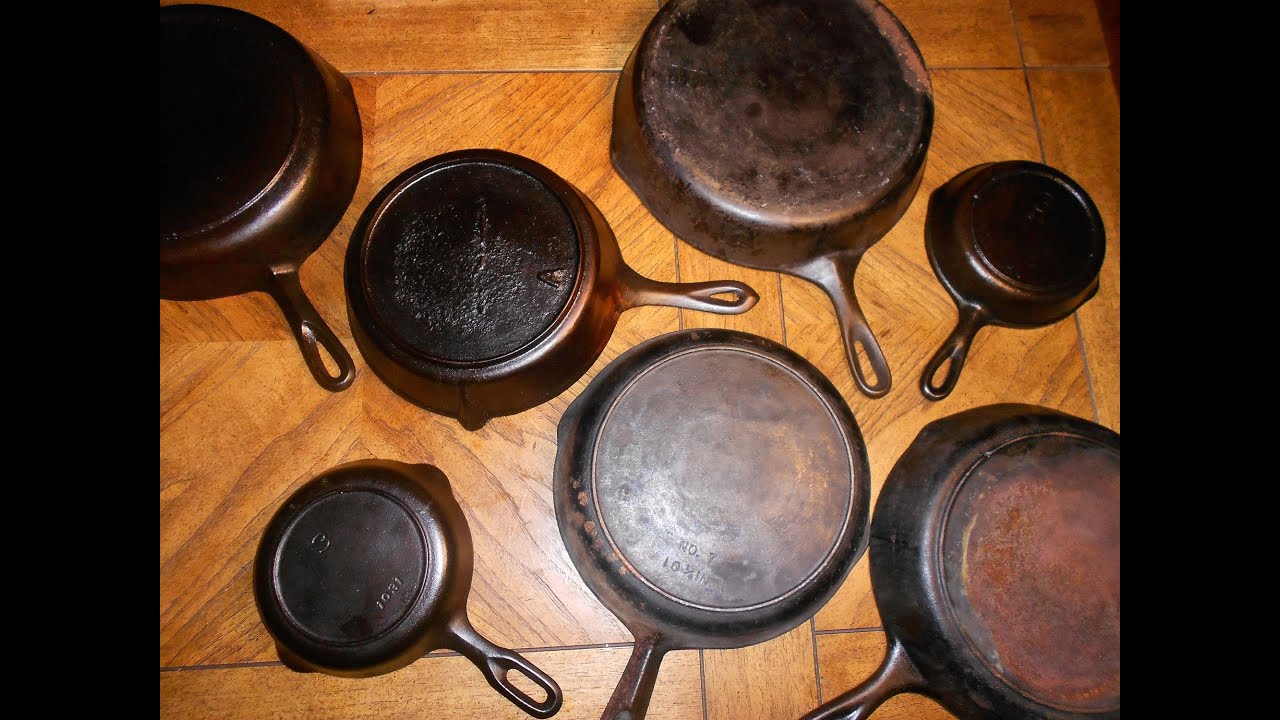This horizontally rectangular, full-color photograph, likely taken indoors with artificial light, displays an array of cast iron skillets of various sizes, all turned upside down, revealing their bottoms. The skillets, which are black and shiny as if oiled and polished, lie on a composite brown surface made up of highly polished wood panels with visible grain patterns. Some of the skillets feature more blackening and signs of use than others, with variations from solid black to burnt reddish-brown tones. Each skillet handle, seamlessly integrated with the pan itself, ends in an oval-shaped hole for hanging. The image is framed with narrow black vertical borders along the left and right edges. The photograph, clearly staged, captures the intricate details of the skillets’ textures and the polished wood beneath them.